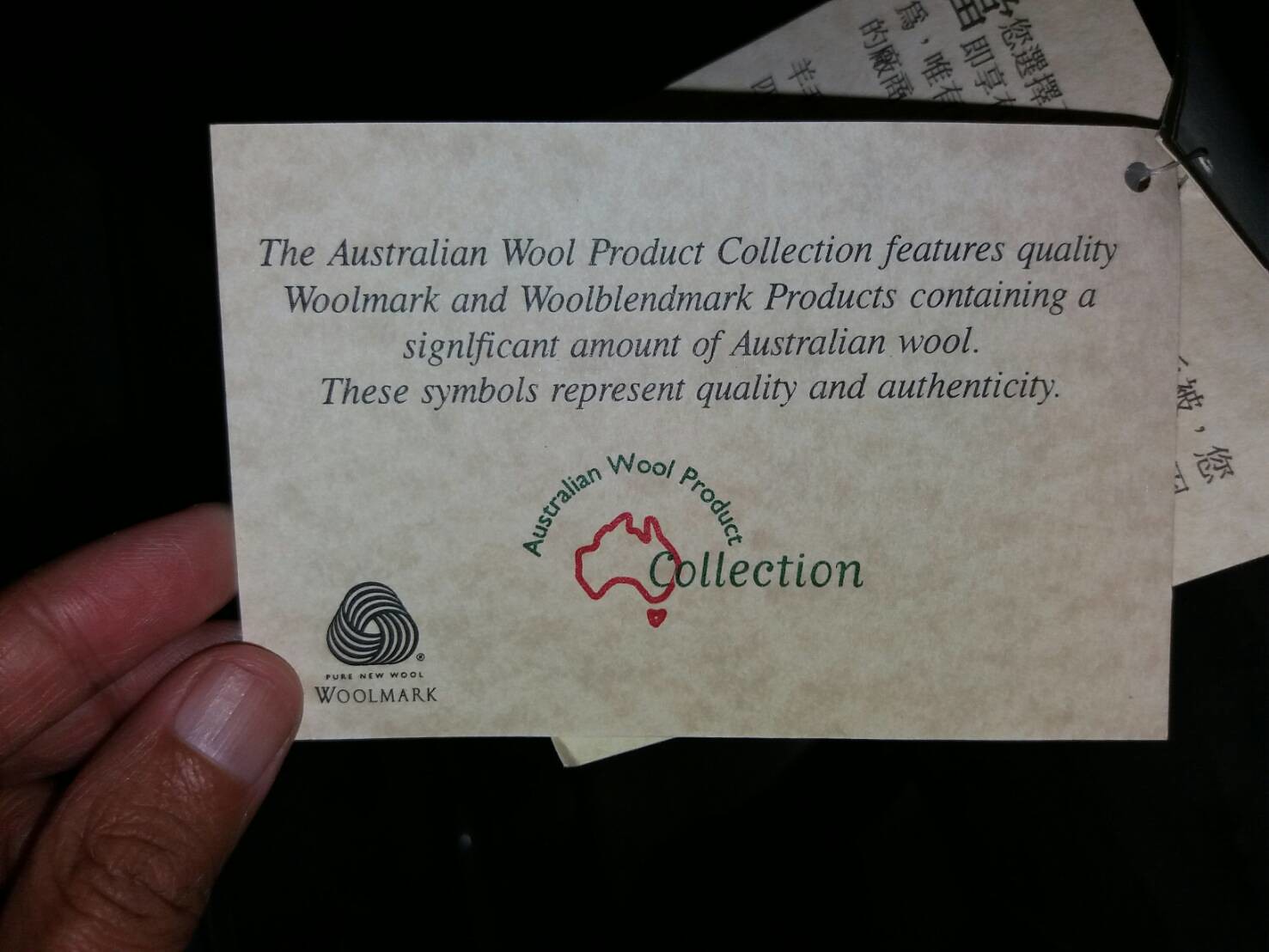The image depicts a left hand holding up a card against a black background. Only three fingers of the hand are visible, with one fingernail showing while the other fingers are turned away. The card has a grayish background and contains black text that reads: "The Australian wool product collection features quality wool mark and wool blend mark products containing a significant amount of Australian wool. These symbols represent quality and authenticity." Below this text, there is a logo featuring the outline of Australia along with the words "Australian wool product collection." At the bottom left corner of the card, the label "Wool Mark" is visible. Additionally, there is a piece of paper below the card, also gray in color and featuring Chinese text.